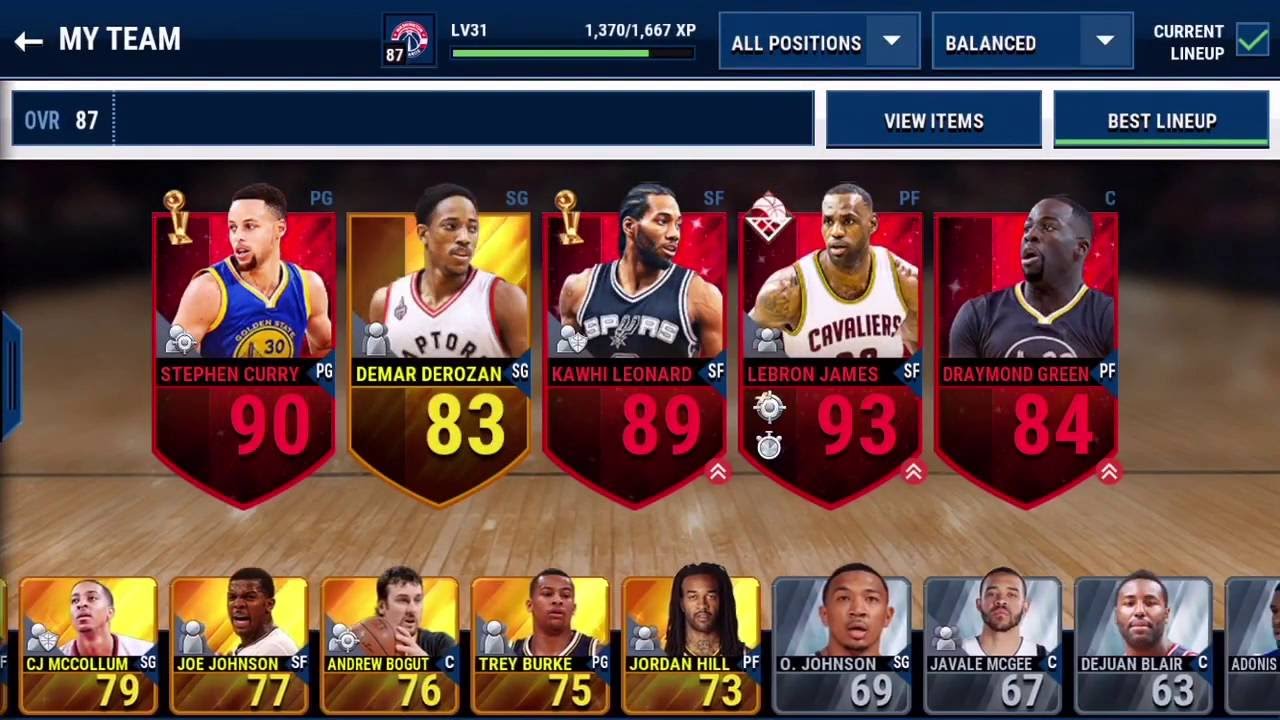This detailed caption describes the My Team screen in the NBA 2K franchise:

"This screenshot captures the My Team screen from the NBA 2K franchise. Dominating the top of the interface, the header is a dark blue with 'My Team' prominently displayed in large white letters on the left side. To the left of the title, there is a left-pointing arrow. On the opposite end of the header, the user's profile photo is displayed, marked with their overall number, '87,' at the bottom right of the icon. Adjacent to the profile icon is a progress bar. At the top left corner of this bar, the user's current level, '31,' is noted, while the XP count is detailed to the right: '1370/1667 XP to the next level.'

To the right of the progress bar, two blue drop-down boxes are present. The first is set to 'All Positions' and the second to 'Balance.' In the far right top corner, the screen indicates 'Current Lineup' alongside a checkbox ticked with a green checkmark. Below this, the text 'OVR 87' denotes the overall rating, next to a blank rectangular bar.

On the far right, there are two prominent buttons, 'View Items' and 'Best Lineup,' the latter highlighted with a green underline. Central to the screen is the lineup featuring superstar players: Stephen Curry, DeMar DeRozan, Kawhi Leonard, LeBron James, and Draymond Green. Below this lineup, eight thumbnails of additional players are fully visible, with partial thumbnails peeking in from the far left and right edges of the screen."